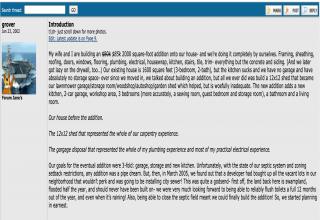This image displays a portion of a website, which appears small and difficult to fully discern due to its size. At the top, there is a prominent blue bar spanning the width of the page. Below this bar, there is a partially visible picture depicting what seems to be a boat navigating through water, with a potential figure situated at the front. The image has a dark, washed-out, and faded quality, making details hard to distinguish.

Directly beneath the image, the word "Introduction" is clearly visible, accompanied by a line of black text, followed by a segment of underlined blue text. The blue text matches the color of the top blue bar. The body of the site contains several paragraphs of black text on a gray background. Some sentences are short, while others are more extended in length. Towards the bottom of the displayed portion, there is a smaller paragraph.

The top blue bar also contains three small boxes aligned to the right; however, due to the size and resolution of the image, the contents of these boxes are indiscernible.